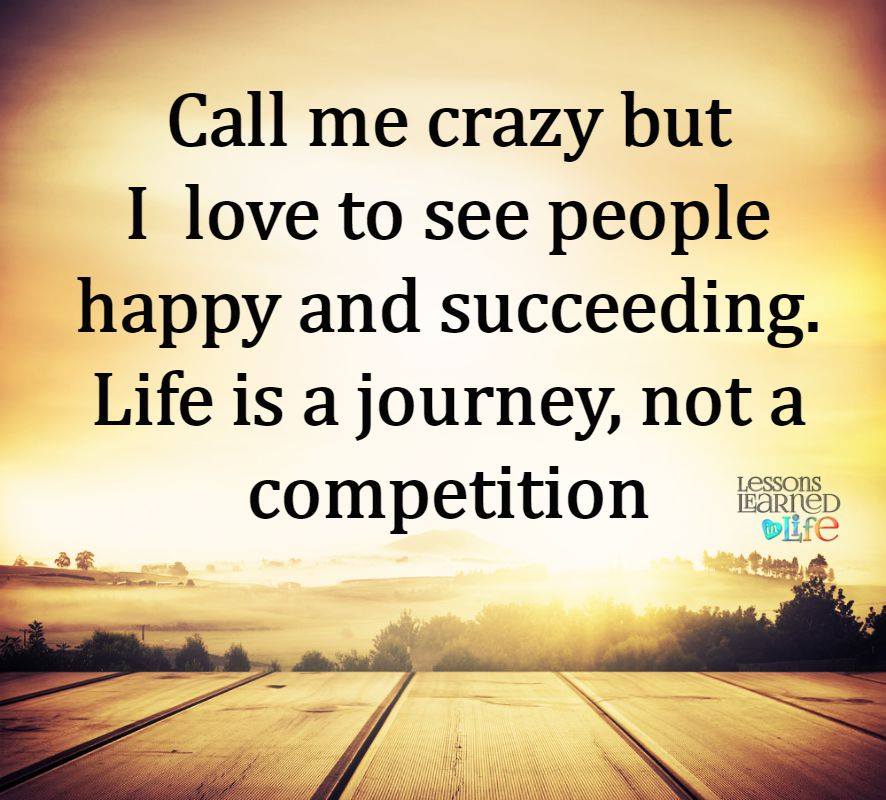The image is a detailed and photorealistic drawing presented as an inspirational panel or plaque. It offers a first-person perspective of standing on a wooden deck or porch, with brown wooden slats extending laterally. The viewer looks out onto a serene landscape where a clear sky is brightened by the rising sun, casting a corona of white, yellow, and brown rays that wash out most of the scene, symbolizing the dawn of a new day. The landscape features a rich array of trees in the foreground, a field, and distant mountains on the horizon, with a barn visible near a hilltop to the right. Overlaying this picturesque scene is a headline in black text that reads, "Call me crazy, but I love to see people happy and succeeding. Life is a journey, not a competition." To the right of this, in smaller print, is the logo "Lessons Learned in Life," with the word "Life" in blue and orange. The overall style merges photographic realism with typographic elements to create an inspiring visual message about life's journey.